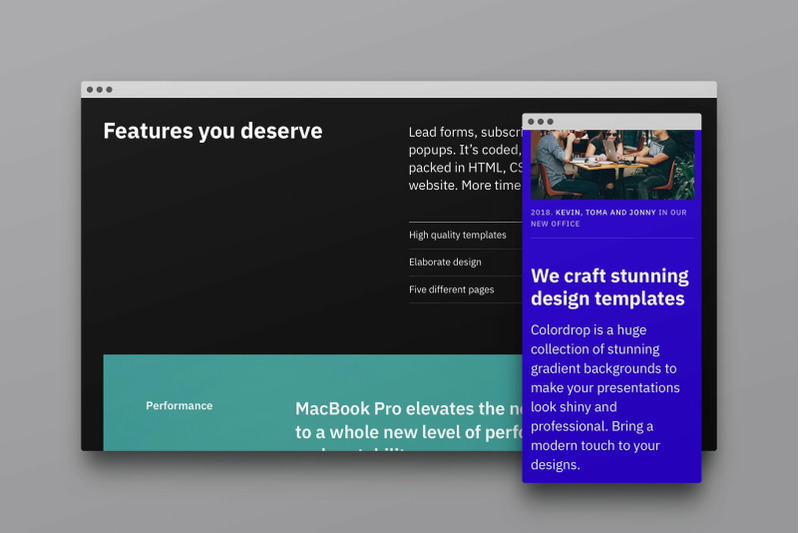In this rectangular image oriented horizontally, we see a solid gray background. Centered within this main frame, there is a smaller, nested rectangle with a black background. Overlaying this black rectangle is a smaller blue rectangle, which appears to be a screenshot from a phone. On the left side of the black background, a bold white text reads "Features You Deserve." Below this, partially covered sentences can be deciphered to include phrases like "lead forms," "pop-ups," "it's coded," "packed in HTML," "website," "more time," and "high-quality templates." These fragmented sentences are separated by a light gray horizontal line, and more words such as "elaborate design" and "five different pages" are visible. In a green area at the bottom of the black rectangle, white text states, "Performance MacBook Pro elevates to a whole new level of." The overall composition suggests a promotional or informational graphic likely related to web design or technology.